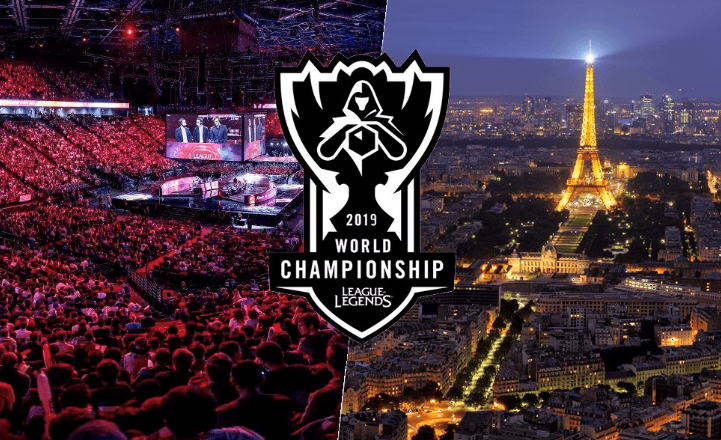The image is a promotional header for the 2019 World Championship for League of Legends, an online multiplayer game. The composition is divided into two halves flanking a central logo. In the middle, the logo displays "2019 World Championship League of Legends" over a trophy-shaped background featuring a hooded figure holding a cube with a sliver of white, symbolizing the League of Legends logo. 

The left side of the image showcases the interior of a packed coliseum bathed in reddish-purple light, with enthusiastic spectators in the stands facing a central stage where gamers compete on their computers. A large four-sided screen above the arena allows attendees to follow the action. 

The right side presents a high-angle nighttime view of Paris, centering on the illuminated Eiffel Tower with a white beacon of light shining from its peak. The Parisian skyline, dotted with buildings and streets, is vividly illuminated against the night sky. This juxtaposition likely indicates that the event took place in Paris, blending the grandeur of the venue with the iconic cityscape.